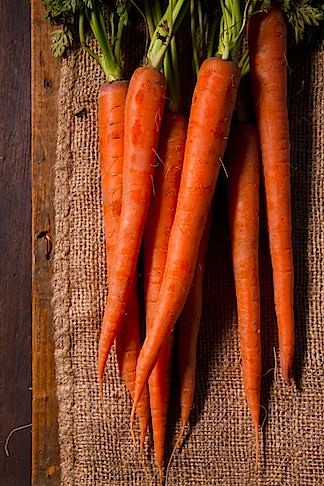This high-quality, top-down photograph showcases a rustic and freshly harvested assortment of seven long, unpeeled carrots. The vibrant orange carrots, complete with their full green stems and fine root hairs at the tips, are arranged in a slightly overlapping vertical formation. They rest on a piece of brown burlap, enhancing the rustic, country feel of the scene. The burlap fabric in turn is laid out on a dark wooden table, adding to the old-fashioned charm of the setting. The professional composition of the image emphasizes the fresh, homegrown nature of the carrots, while the cropping just lightly trims the tops of the green stems, keeping the focus on the earthy vibrancy of the vegetables.